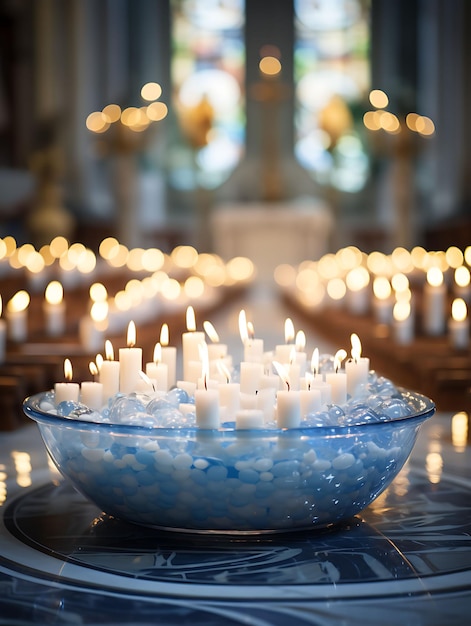The image depicts the interior of a church or cathedral, characterized by its blurred stained glass windows in the background. Central to the composition is a transparent glass bowl with a subtle blue tint, filled with an assortment of clear marbles and white pebbles. Nestled among these decorative elements are several small, white pillar candles, all of which are lit and give off a warm glow. The bowl is placed on a highly polished, possibly marble, ornate table that adds an element of sophistication to the scene. The background, though blurred, reveals additional lit candles and the faint outline of wooden pews, contributing to the sacred and serene atmosphere. The overall bright lighting enhances the clarity and vividness of the scene, emphasizing the bowl of candles as the focal point.